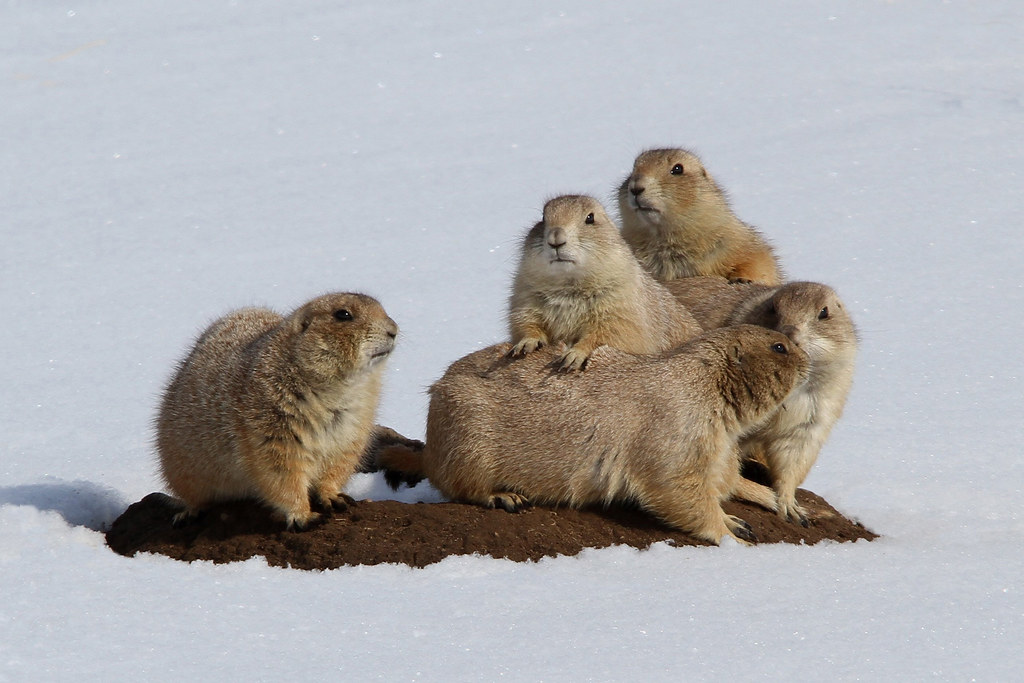The photo captures five rodent-like animals, most likely prairie dogs or possibly gophers, huddled together on a small patch of freshly dug brown dirt. Surrounding them, the entire background is covered in snow, creating a striking contrast with the bare ground. These rodents all have light brown, almost beige fur and black eyes. They are of similar size and appear quite large for rodents. In the scene, one animal on the left looks cautiously at the camera. The two in the center face different directions, with one standing on the other's back. On the far right, two animals are looking directly at the camera, one standing behind the other with its paws resting on its companion's back. The composition highlights the small snowy world these curious and social creatures inhabit, with their mound of dirt measuring roughly three feet long and a foot and a half wide as the only refuge from the snow-covered surroundings.